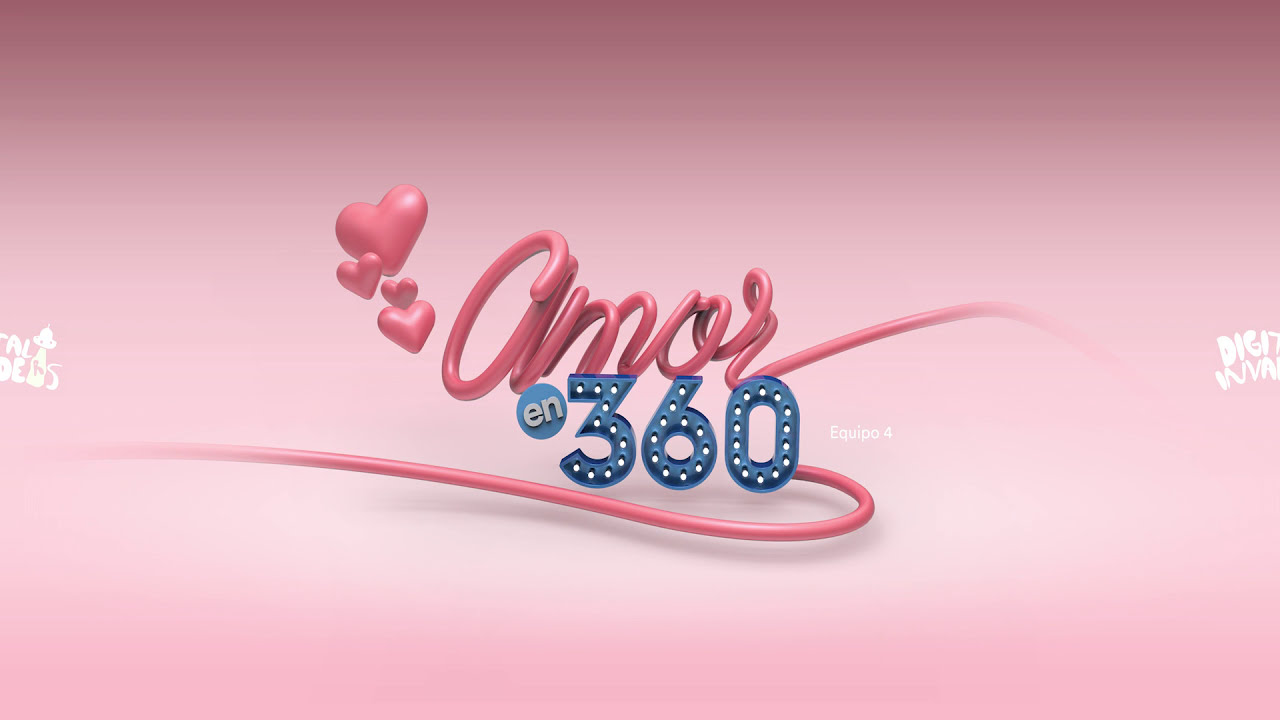The image features a company logo centered against a predominantly pink background with various shades, transitioning from darker pink at the top to a lighter pink towards the bottom. In the center of the image, the word “Amor” is displayed prominently in a dark pink, script-like font made to resemble a windy, plastic string, with the string extending to the right and partially beneath the letters. Directly below "Amor" is the number "360" in blue, with "E-N" in silver-white within a blue circle adjacent to it. To the left of "Amor," there are four pink hearts of varying sizes aligned vertically above the letter "A." On the far right side of the image, partially obscured, are the white letters "D-I-G," suggesting the beginning of a word like "Digital." Additional unclear lettering appears faintly on the left and right sides of the image. The overall design gives the impression of a digital logo, possibly intended for a company website, emphasizing themes of love and inclusivity with its pink, heart-laden aesthetic.